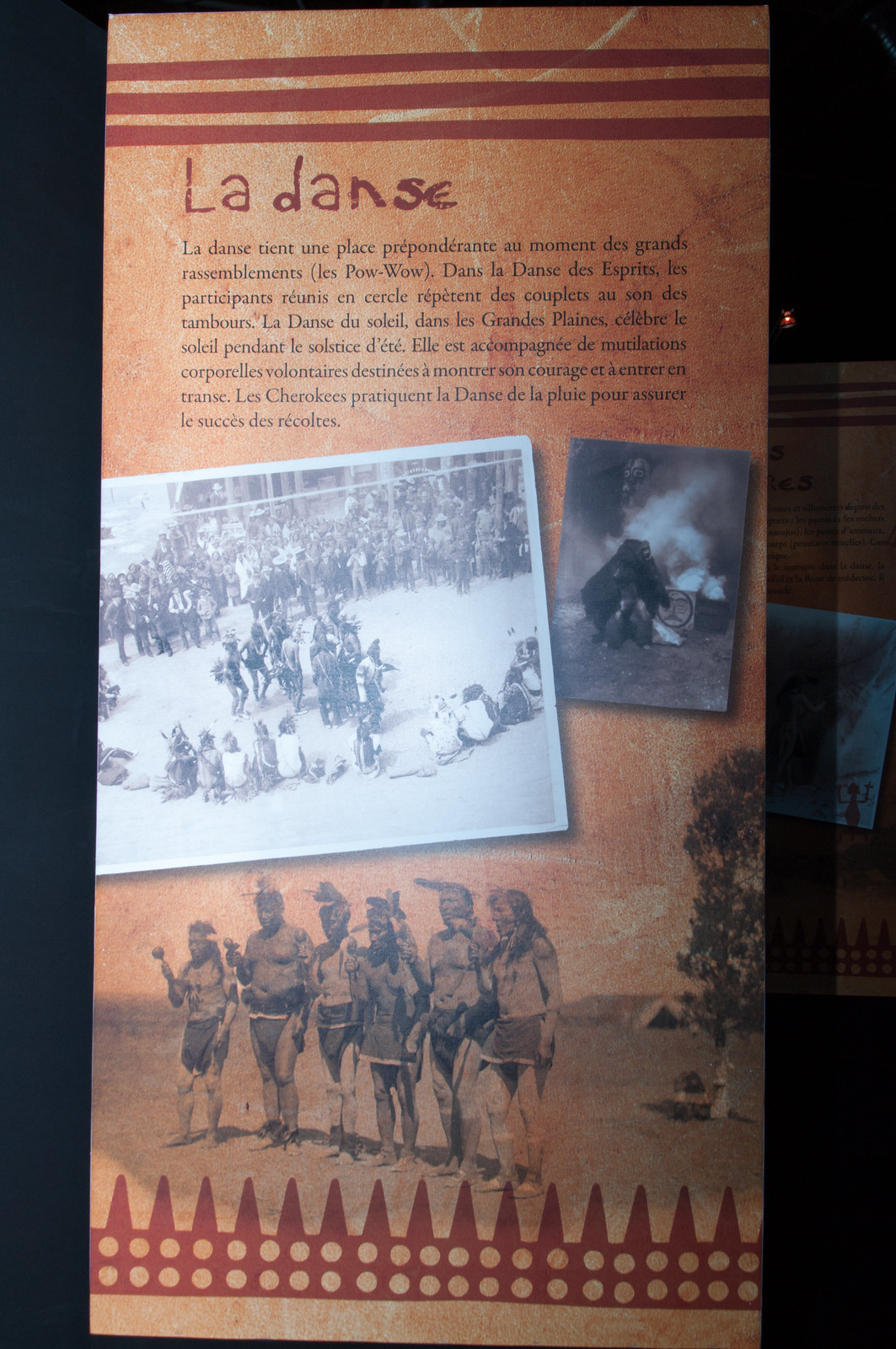This image appears to be an excerpt from a textbook or a museum display, presented on a background of brownish-red color. At the top, the title "La Dance," written in bold red letters, seems to introduce the subject matter. Below the title, there's a paragraph written in French, consisting of approximately eight lines, though the text itself is too fine to read clearly. Beneath this paragraph is a black and white photograph showing people seated in a circle, with others performing in the center, suggesting some form of dance or performance, likely a cultural or celebratory event involving Native Americans. To the right of this scene is another image, which appears to depict a cannon firing. At the bottom of the display, a group of Native Americans is shown standing in a row, adorned with feathered headdresses and holding objects in their right hands, possibly participating in a traditional dance. A small tree is visible on the right-hand side of this lower section, accompanied by an intricate geometric design featuring triangles and circles. The details point toward the display being an informative piece about Native American traditions, particularly their dance ceremonies and powwows.